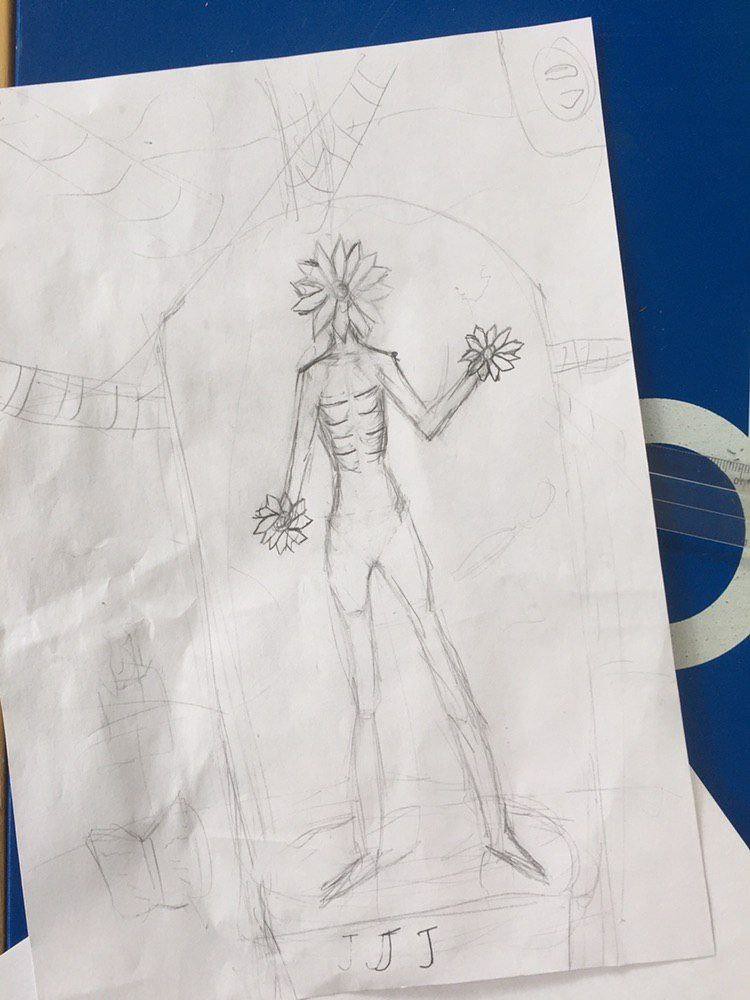This image showcases a pencil sketch set against a royal blue background with white accents, possibly resembling a pinboard or tabletop. The blue backdrop might also feature a ruler along the edge. At the center of the image lies a single sheet of paper displaying a primitive pencil drawing. The sketch depicts a stick-figure-like human with unconventional flower petals replacing the face and hands. This rudimentary figure is situated within an arch-like structure, from which lines emanate, possibly suggesting support. Beside the figure is a roughly drawn image of a book. Along the bottom of the sketch, the letters "J, J, J" are inscribed.